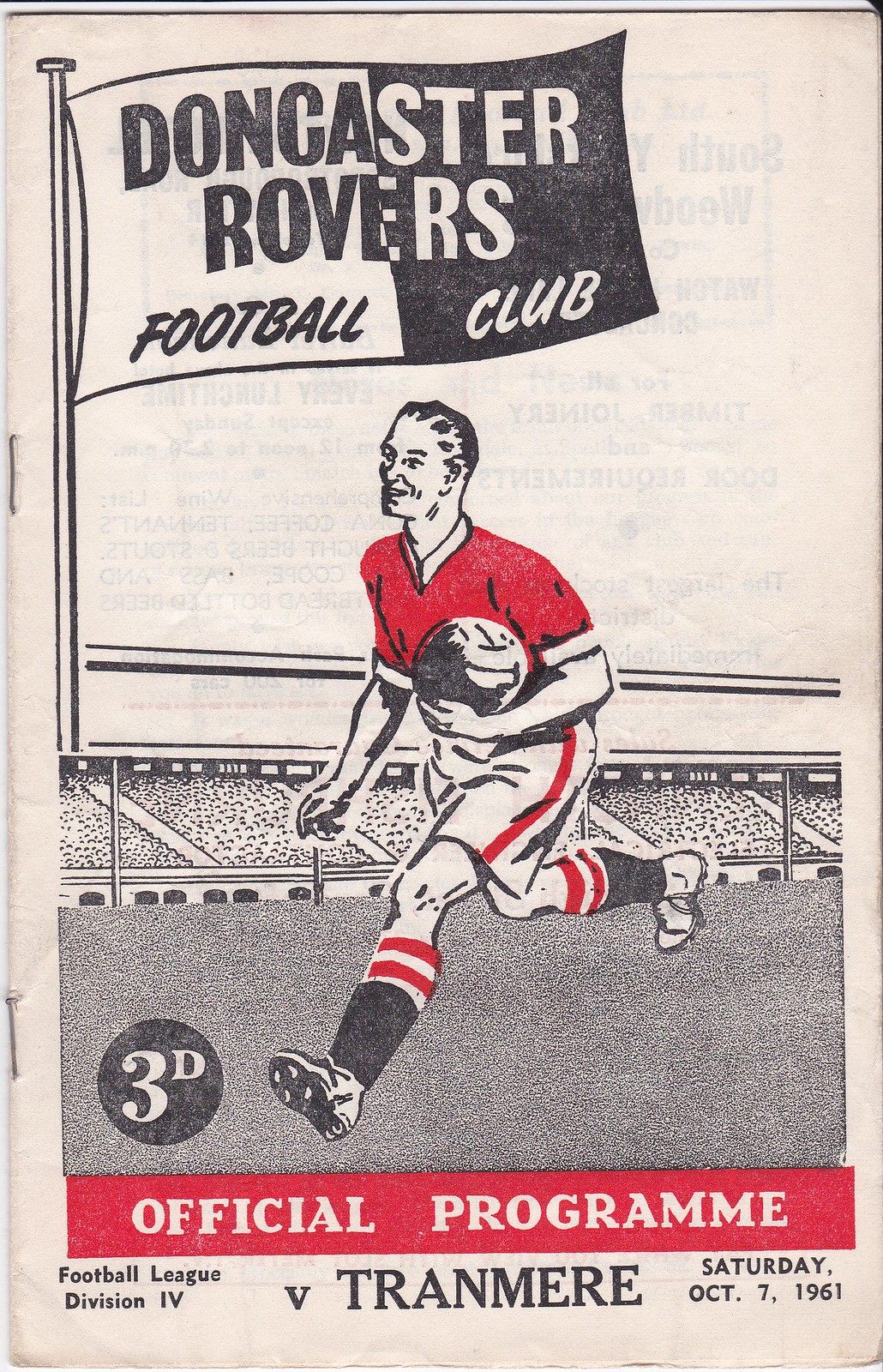This rectangular image, resembling the front cover of an old magazine, measures about six inches tall and three inches wide. It is held together by two staples on the left-hand side. The background color is a faded yellowish pink, reminiscent of aged newspaper. Dominating the top left corner is a flagpole with a flag that reads "Doncaster Rovers Football Club," split vertically with white on the left side and black on the right, and featuring alternating black and white print.

Below the flag, a cartoon illustration depicts a man in mid-run, holding a round soccer ball in his left hand. He sports a red short-sleeve shirt, white shorts with a red stripe down the side, and black socks capped with white and red. His dark hair and visible football shoes complete his animated look, and he appears to be running past a stadium filled with spectators.

In the lower left-hand corner, a black circle with white text reads "3D." Directly beneath the illustration is a red banner with "Official Program" written in white letters. Further down, in smaller black text, it states "Football League Division 4 v. Tranmere," followed by the date "Saturday, October 7th, 1961" in the bottom right corner, confirming the program's historical context. This comprehensive visual captures the excitement and nostalgia of a significant football match from 1961.